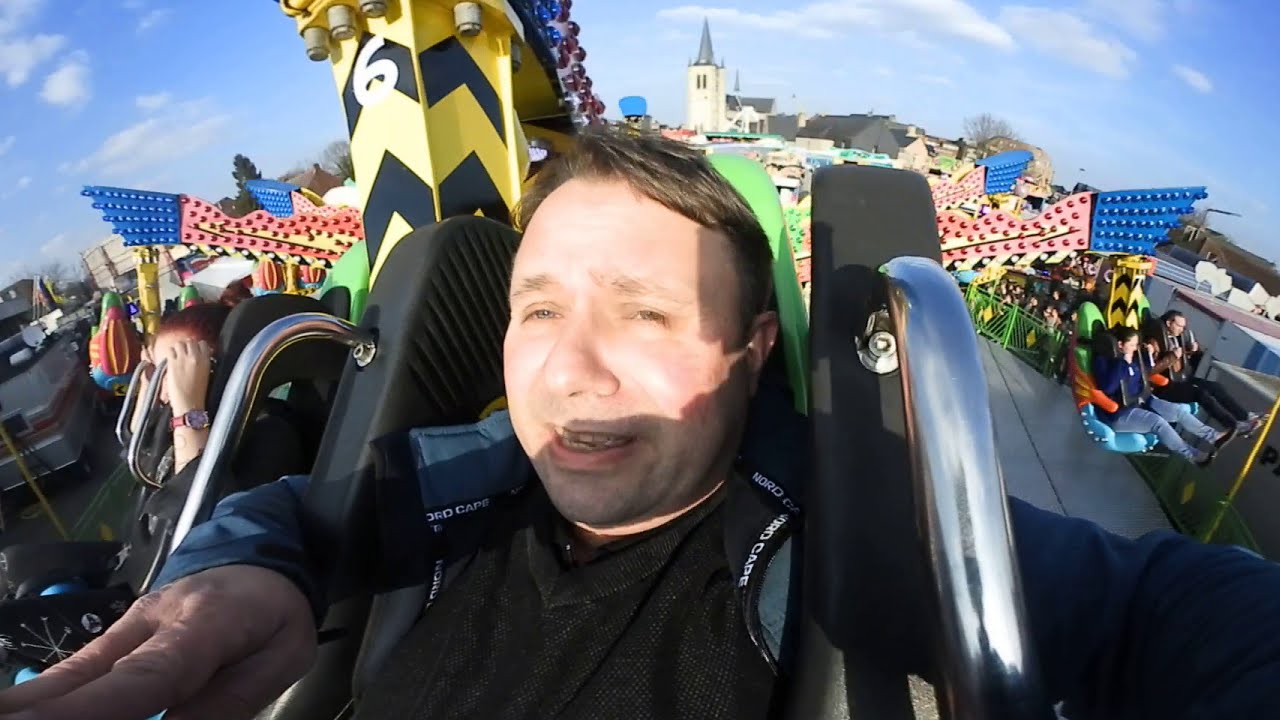In this vibrant and lively image taken at an amusement park on a sunny day, the foreground is dominated by a close-up of a smiling Caucasian man with brown hair, who is seated in a ride seat equipped with metal railings and a seatbelt. He seems to be taking a selfie, capturing his joyful expression. Beside him, to his right, a girl with red hair is also seated, wearing a watch, and smiling. Surrounding them, the scene is filled with other riders whose legs dangle in the air, emphasizing the thrill of the ride. The backdrop of the image showcases an array of colorful elements, including flags adorned with lights and various hues of blue, red, yellow, black, and green that add to the festive atmosphere. The sky is a clear, vivid blue with a few clouds, and a tall spiraled building stands prominently in the background, enhancing the lively carnival or fair setting. The overall composition vividly captures the exhilarating and happy moments shared by the riders.